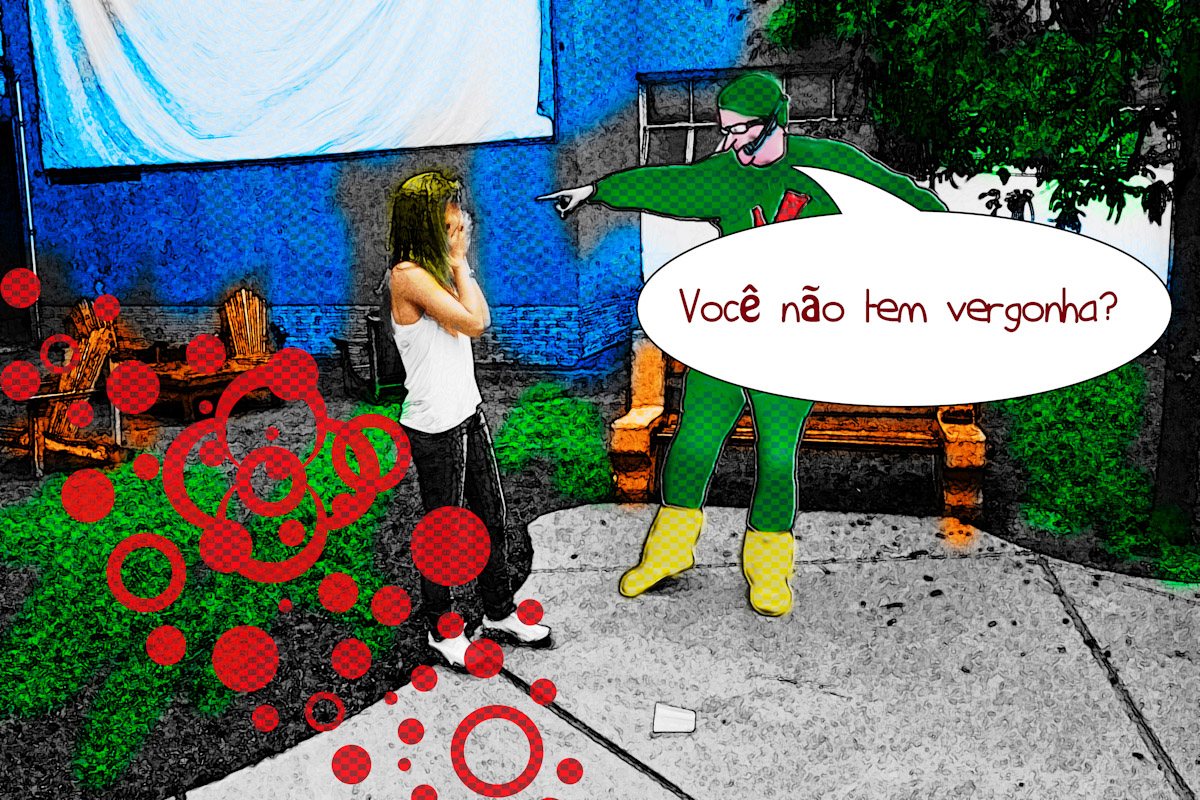The highly edited photograph features a surreal, artistic scene overlaid with a comic filter, rendering everything in a checkerboard pattern. In the foreground, to the left, stands a girl with long dark (or yellow) hair wearing a white tank top, black pants, and white shoes. Her hands are pulled over her mouth, obscuring her face. To the right, a cartoonish man in a green superhero suit with a green helmet and white (or yellow) boots is pointing at her. He holds a microphone close to his mouth and a speech bubble with brown font that reads, "VOCÊ NÃO TEM VERGONHA?" ("Aren't you ashamed?"). 

Behind them, the background showcases a tall, blue building with a white projection screen or sheet draped on the wall. To the right of the building is a tree and some brightly-colored green plants, suggesting a small courtyard or garden. Between the two foreground characters, there are two wooden chairs situated in front of a green shrubbery. Additionally, various red circles of different sizes—some hollow, others solid—are scattered across the image, adding to its surreal and cartoonish aesthetic.